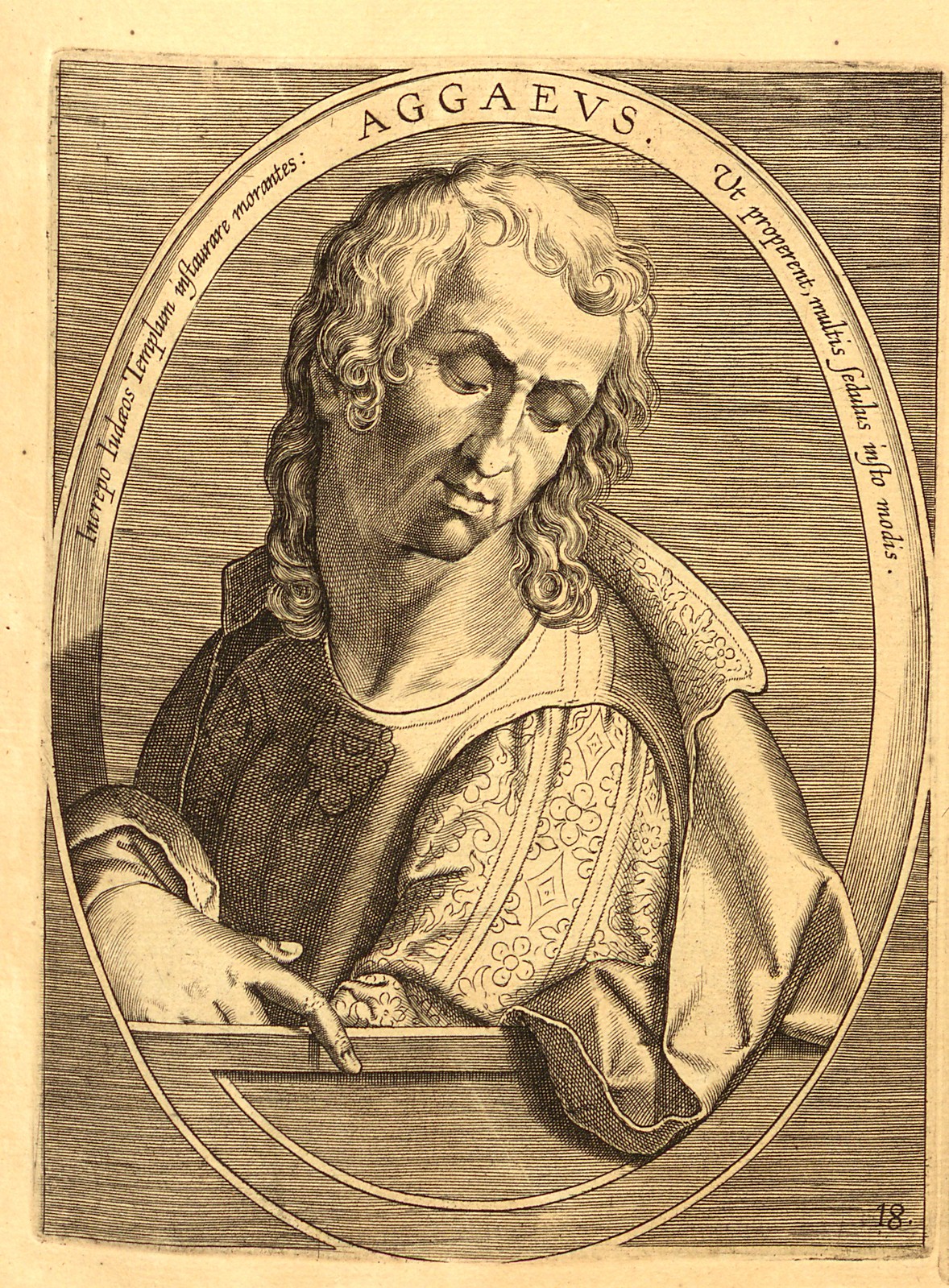The image depicts an old European-style drawing of an older man with shoulder-length curly hair, adorned in priestly or royal garb made of smooth fabric. He is gazing downwards, possibly behind a pulpit or a balcony. The artwork is rendered in black ink on yellow, aged paper, and is encased within an oval boundary. Surrounding the drawing is Latin text: “Increpo Iudios Templum Inflorentre Morantes” on the left and “Ut Properent Multis Fedulis Info Modis” on the right. Above the man's head, the word “AGGAEVS” is inscribed. The background of the image features narrow horizontal black lines, giving it a striped appearance and adding to the overall antiquated feel of the piece.